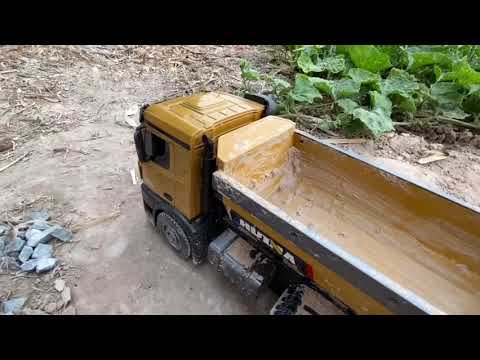The daytime outdoor photograph captures a yellow dump truck with a black stripe along the dump bed and the letters "MUINA" on its side. The dump truck is positioned slightly towards the upper left and is viewed from an elevated angle. Its bed is empty and dirty, with the back gate lowered, and the windows appear open, revealing an unoccupied cabin. The truck's large, mud-covered wheels rest on a ground dominated by brown dirt, with patches of dried-out grass, sticks, and weeds scattered around. To the truck's left is a small pile of granite rocks, some gray with white portions. On the right side of the image, large green leaves reminiscent of collard greens are visible. A notable feature of the photograph is the black bars running horizontally across the very top and bottom edges of the image.